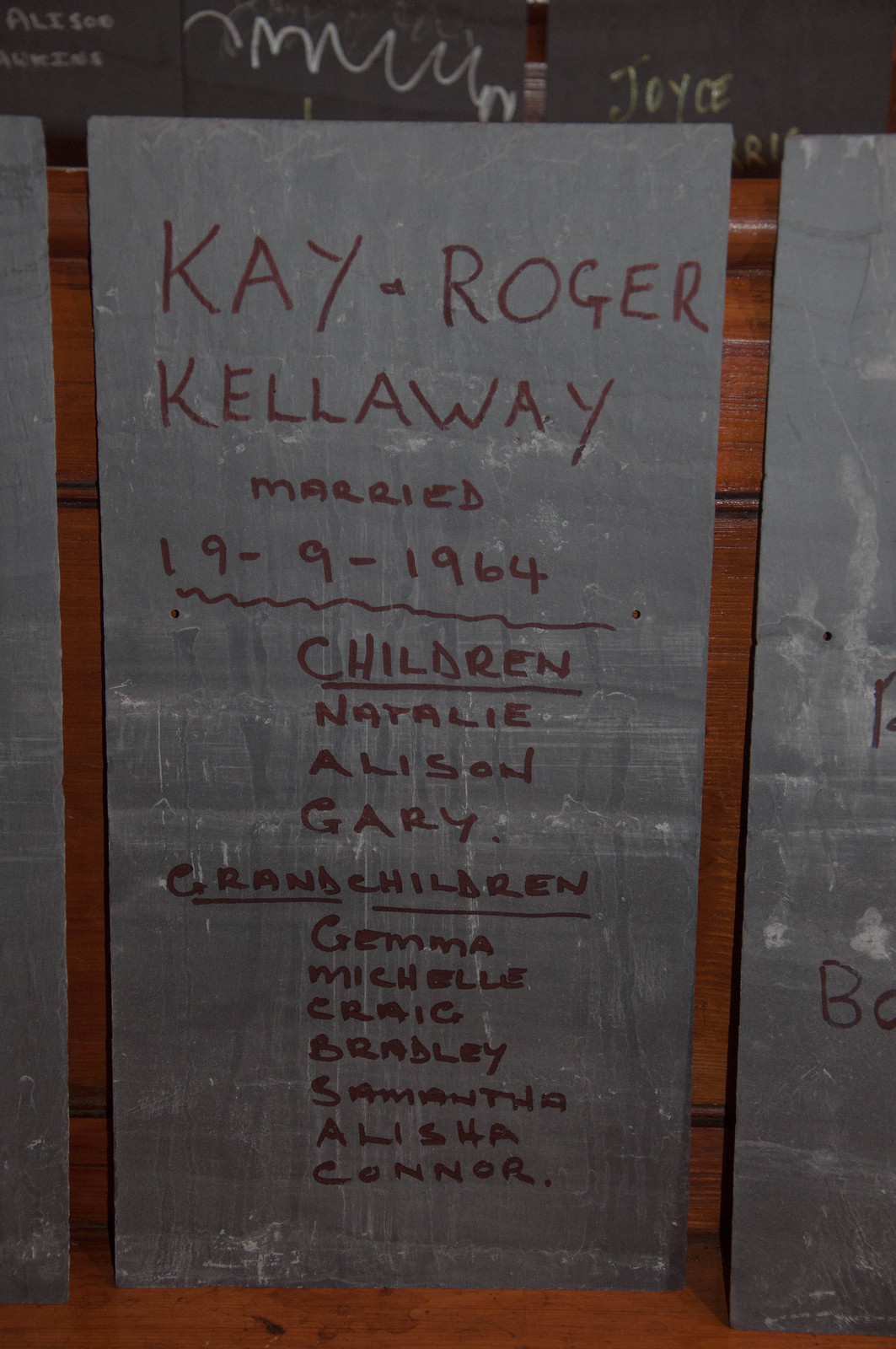The image depicts a handwritten sign, possibly made from either gray slate, plastic, or tin, featuring information about Kaye and Roger Kellaway. The sign, vertical in orientation and central to the image, commemorates their marriage from 1909 to 1964. Written in black marker or ink, it lists their children—Natalie, Allison, and Gary—and their grandchildren—Gemma, Michelle, Craig, Bradley, Samantha, Alicia, and Connor. The text includes underlined headers for "CHILDREN" and "GRANDCHILDREN," both followed by squiggly lines. The sign leans against a brown wooden background, with additional similar signs visible but partially obscured. The overall color palette consists mainly of gray tones for the slate or plastic and brown for the wood. There are holes punched in the sign, suggesting it might be designed to hang.